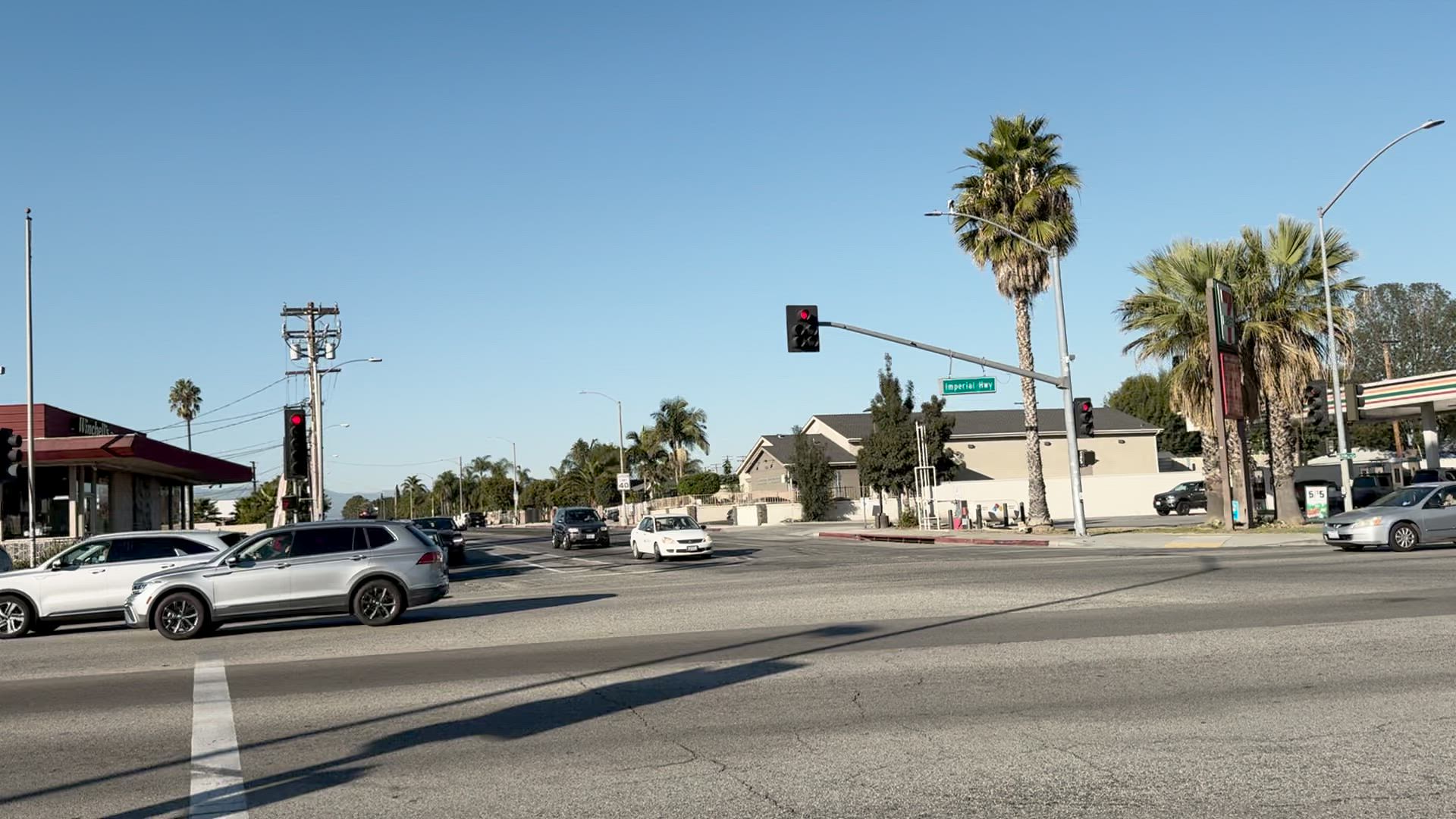A vibrant daylight captures an outdoor scene at a busy four-way intersection, viewed from a slightly diagonal perspective. In the lower left to lower right part of the image, a two-lane road spans across, with traffic moving from left to right in the far background lane. This lane includes two SUVs on the left and a silver sedan just entering the frame from the upper right. Perpendicular to this road, another stretches diagonally to the left and out of sight, where two cars are waiting.

The traffic light, central to the photograph and showing a red signal, is mounted on a post on the sidewalk to the right, behind which stands a tall palm tree. The upper half of the image is dominated by a clear blue sky. On the left side in the background, part of a building’s facade is visible along with a utility pole bearing two transformers.

In the far right corner, an awning of a gas station is observable beside two more palm trees situated in the foreground. The lower third of the image is filled with the gray macadam of the street, displaying a shadow or reflection of a street sign that stretches diagonally from the lower left, indicating the Sun's position from the foreground to the left. The photograph is free from any visible text or print.